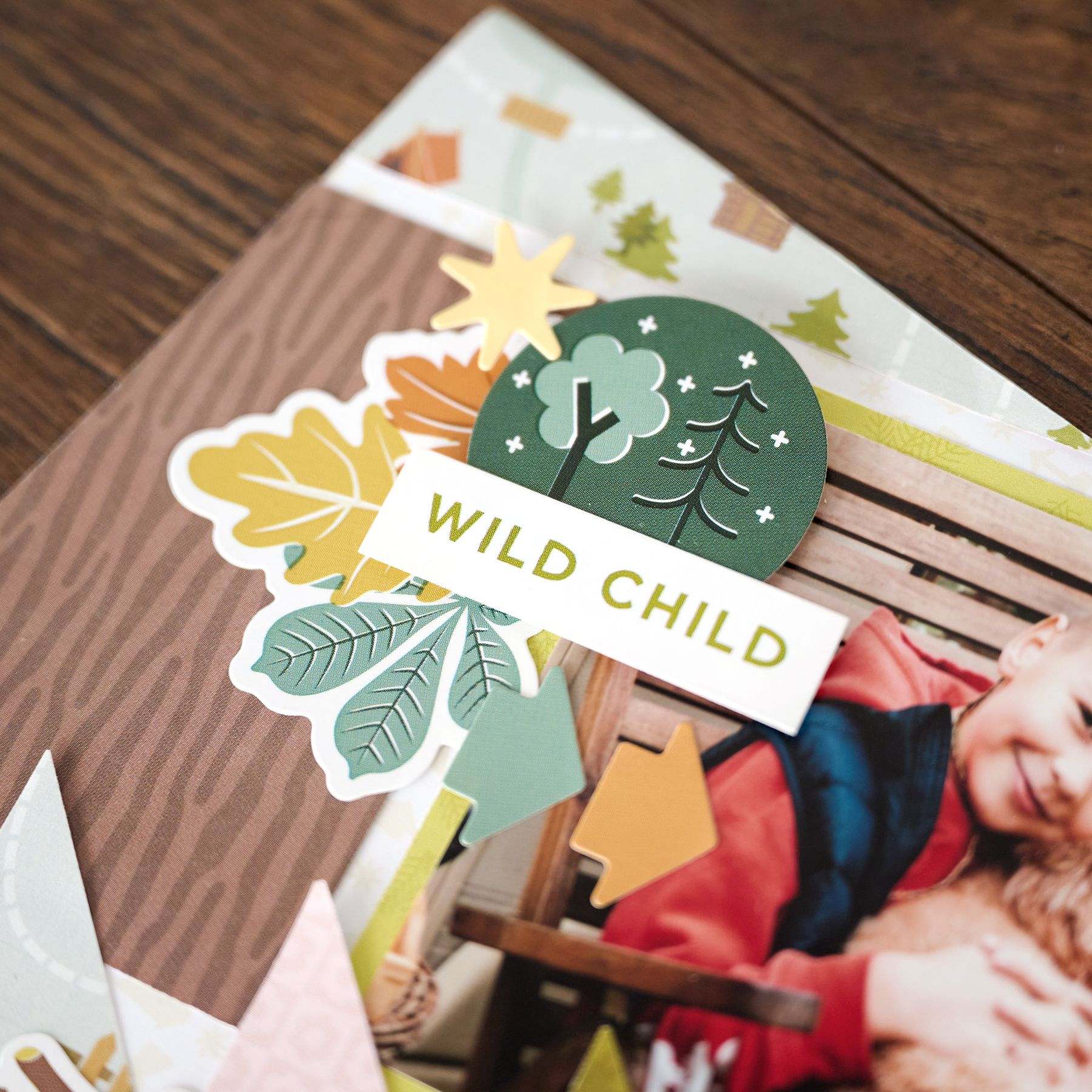The photograph showcases a meticulously crafted scrapbook placed on a dark brown wooden table. The focal point of the scrapbook is a picture of a young boy, around five years old, with short blonde hair, wearing a red jacket with a black vest over it. He is lovingly hugging a light tan, shaggy dog while seated on a brown wooden chair. Above and around this photograph are various decorative elements, including a green circular sticker with two trees, a white block with green lettering that says "Wild Child", and an assortment of leaves in orange, yellow, and green hues, enhancing the outdoor theme. The background pages of the scrapbook feature a white one adorned with pine trees, campsites, and tents, and another with a brown zebra print design. This detailed and vibrant scrapbook page appears to be part of a kit, complete with all the necessary stencils, stickers, and decorations for a personalized, outdoor-themed project.